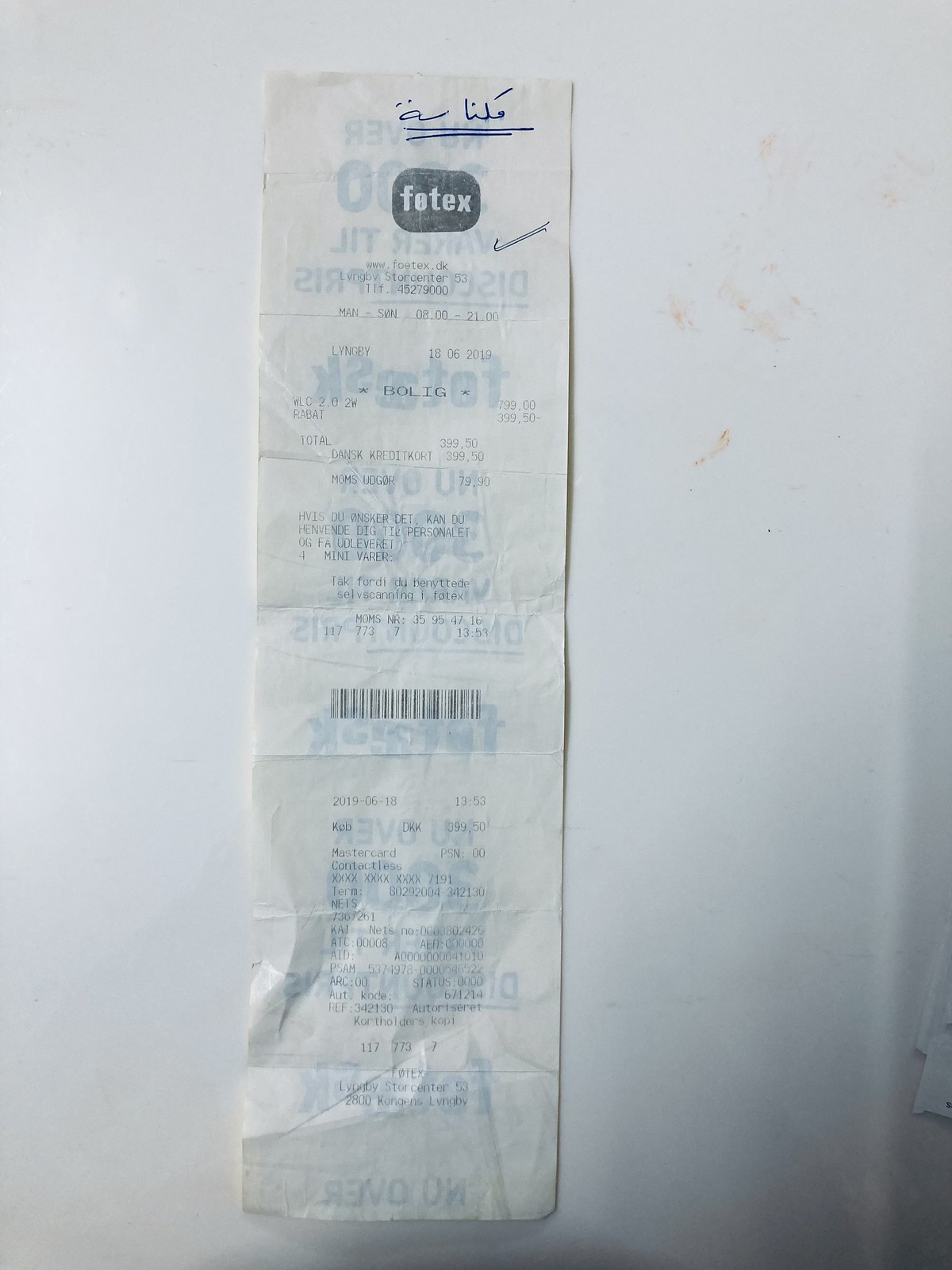This detailed photograph showcases a long receipt from a Danish store named Fotex, identifiable by its black square logo and the website fotex.dk, which confirms its Danish origin. The receipt appears to be double-sided, with text from the back bleeding through, making it challenging to decipher. Handwritten notes at the top in blue pen, underlined twice with two check marks, are present. The items listed are written in Danish, and it's noted that the person paid using MasterCard. The amounts indicated on the receipt include "7.99,00" and "3.99,50" (with the latter showing a negative sign). While the exact details and total amounts are hard to determine due to the text bleeding through, it is clear that this receipt pertains to a purchase made in Denmark, likely at a department store given the context and typical format.